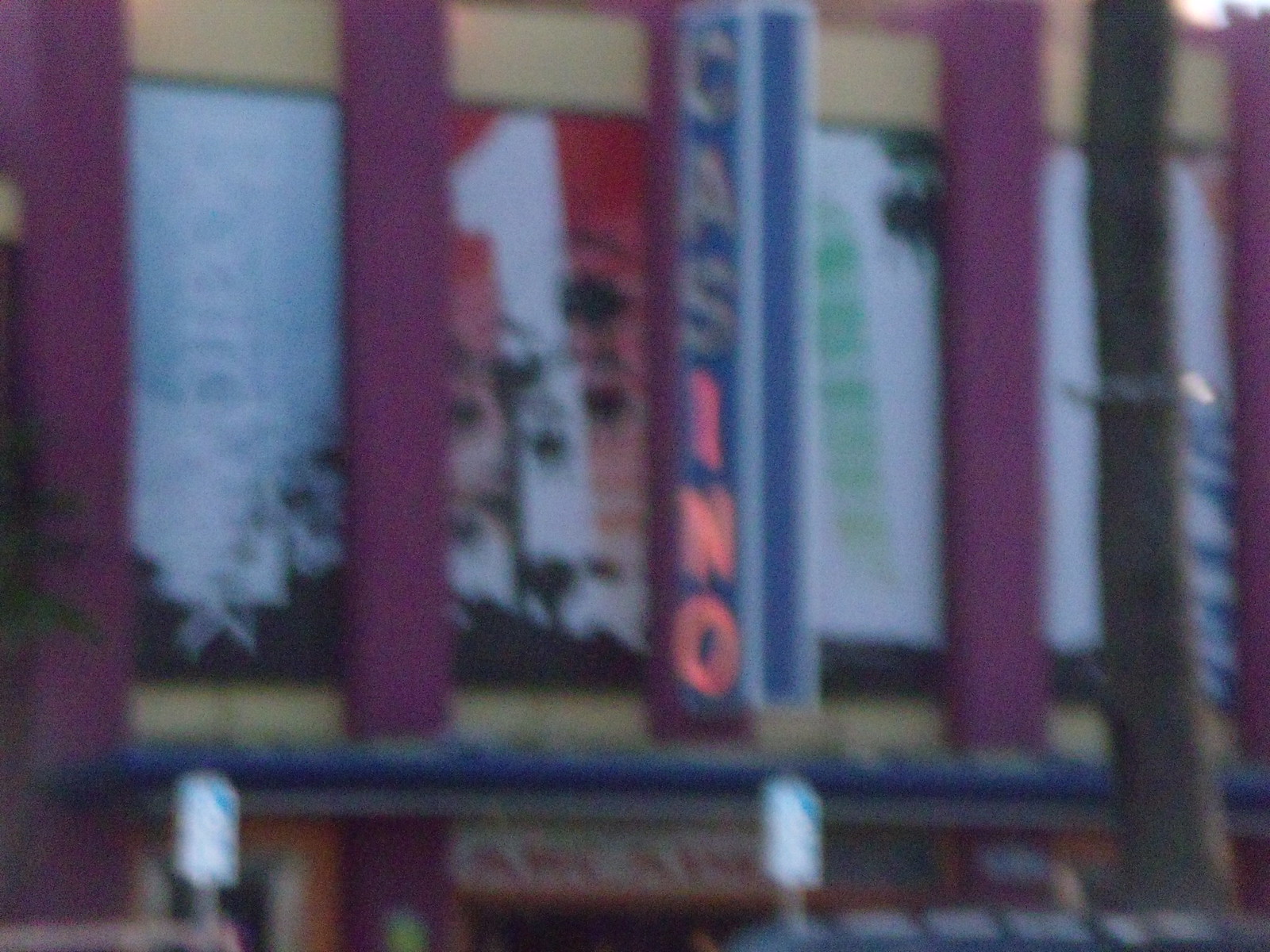The image is a significantly blurry photograph depicting the front of a casino. Overhead, colorful banners in shades of blue, white, red, black, and green hang prominently. In the center, a blue rectangular sign with tan-colored letters spells out "CAS," while the remaining letters "INO" are in bright neon orange. This central sign is attached to the building, flanked by large purple bars. Below this sign, a blue awning is also visible. The building itself has a light tan color, contributing to its muted appearance. Among the several other signs around, one red sign features a large white number "1". Some signs have white lettering on a light blue background, while others have indiscernible green imagery. The foreground of the image shows blurry white and blue handicapped parking signs outlined in the lot. Despite the blurriness, the overall setting gives a vivid sense of a casino entrance adorned with vibrant, though indistinct, decorations.